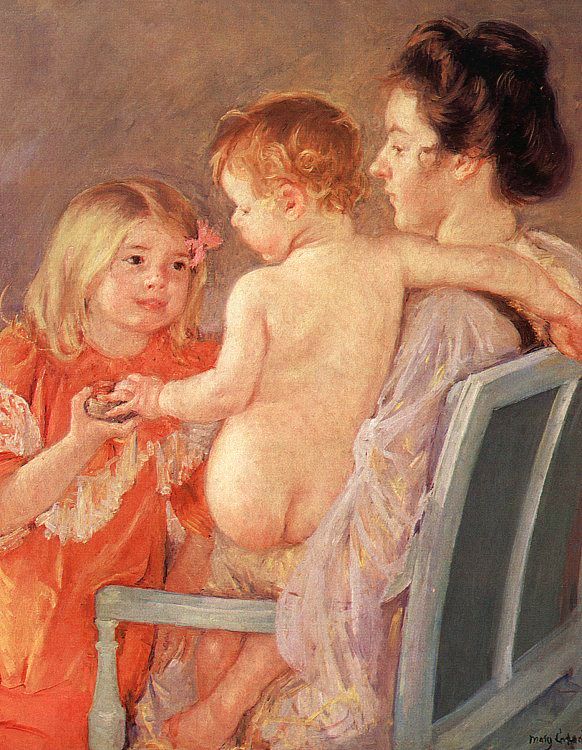This is a vertically oriented Impressionist painting by Mary Cassatt, depicting a tender moment between a mother and her two daughters. The mother, seated on a light blue or grayish bench, looks calmly towards the left. Her dark brown hair is styled in an updo, and she wears a lacy white gown. She holds a naked baby with short, curly reddish-blonde hair on her left hip. The baby is looking towards and holding the hand of an older sister. The baby’s tiny right arm drapes over the mother's shoulder.

The older sister, approximately seven or eight years old, stands to the mother's left. She has shoulder-length blonde hair adorned with an orange flower near her left ear. Her brown eyes gaze lovingly at the baby, and she wears a flowing orange and white robe. The backdrop of the painting is composed of warm brown hues, enhancing the intimate and cozy atmosphere of the scene. In the bottom left corner, partially legible, the artist’s signature reads “Mary C,” likely Mary Cassatt, confirming the artwork’s origin.